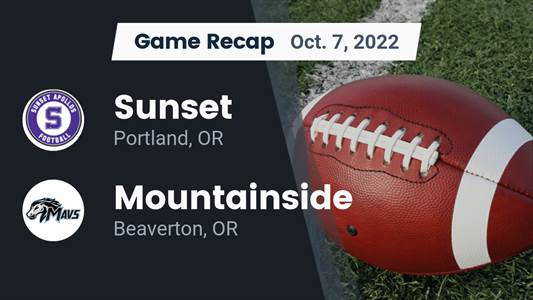This outdoor, photographic image serves as an informational sign for a football game recap, dated October 7th, 2022. The background is predominantly dark gray on the left side and green grass on the right, reminiscent of a football field. The top of the image features a white rectangle with the heading "Game Recap, October 7, 2022." Below this heading, the left section displays the names of the competing teams: "Sunset, Portland, Oregon" and "Mountainside, Beaverton, Oregon." Each team is represented by its emblem, with Sunset's emblem showing a circle with an 'S' labeled "Sunset Apollo's football" and Mountainside's emblem featuring a graphic of a horse and the word "Mavs." Occupying the right section, a large brown football with white lacing and white end bands rests on a patch of grass, complete with white field markings. This visual summary focuses on the football details and team emblems for a clear presentation of the game recap.